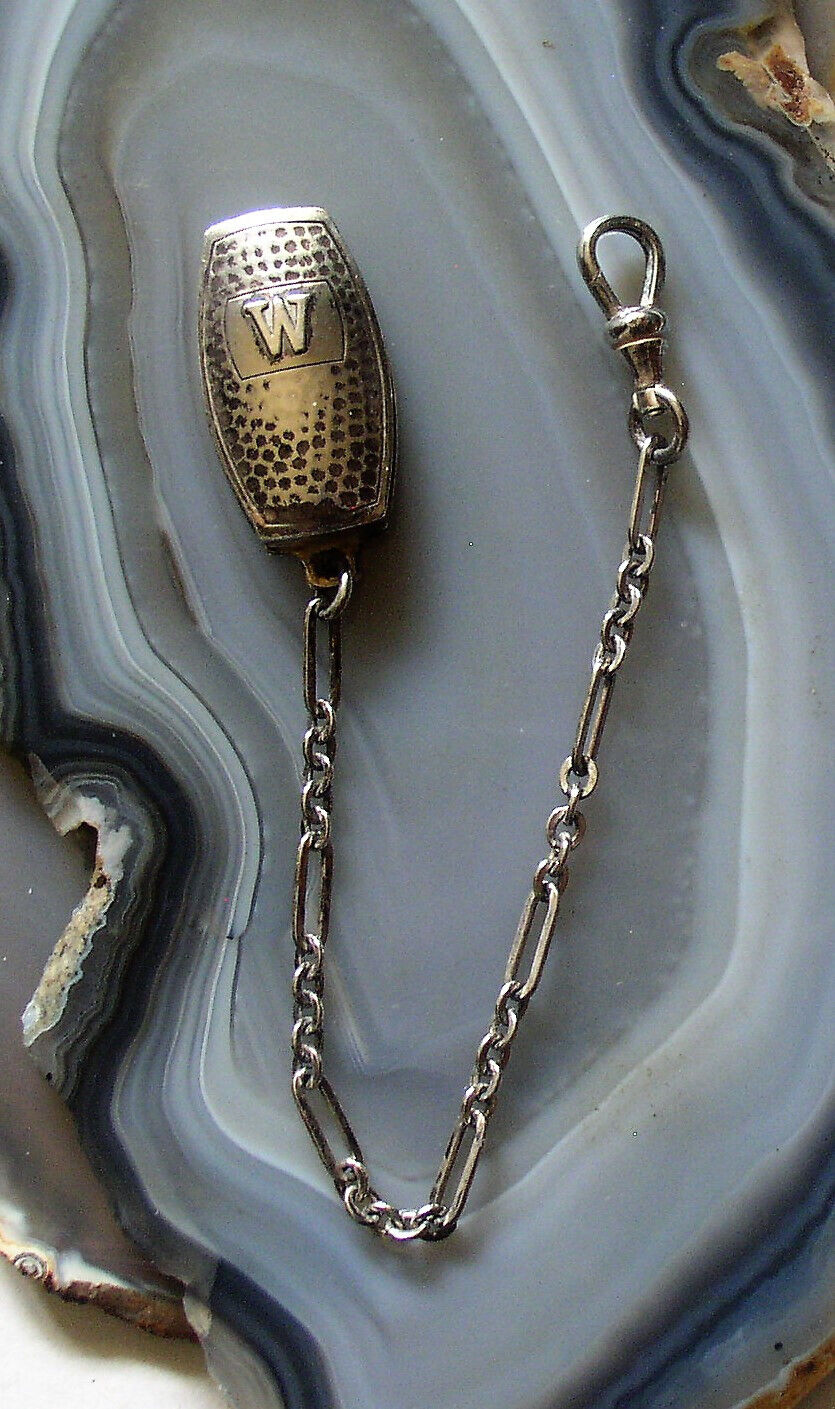The photograph captures a piece of jewelry artistically displayed on a white, semi-oval plate that resembles the inside of an oyster shell, bordered in shades of gray and black, suggesting an authentic oyster-like texture. The centerpiece is a distinctive, small metal device with tarnished, silver-gold tones featuring an inscribed "W" and shaped somewhat like a beer barrel. The metal piece appears perforated with holes and might be capable of being opened. Attached to this device is a gold and silver chain, meticulously detailed with seven interlocking links connected by smaller rings. The chain culminates in a gold loop and clasp, glistening as if nearly new. The intricate positioning on the oyster-like plate enhances the visual appeal, though the overall size remains ambiguous due to the lack of surrounding context.